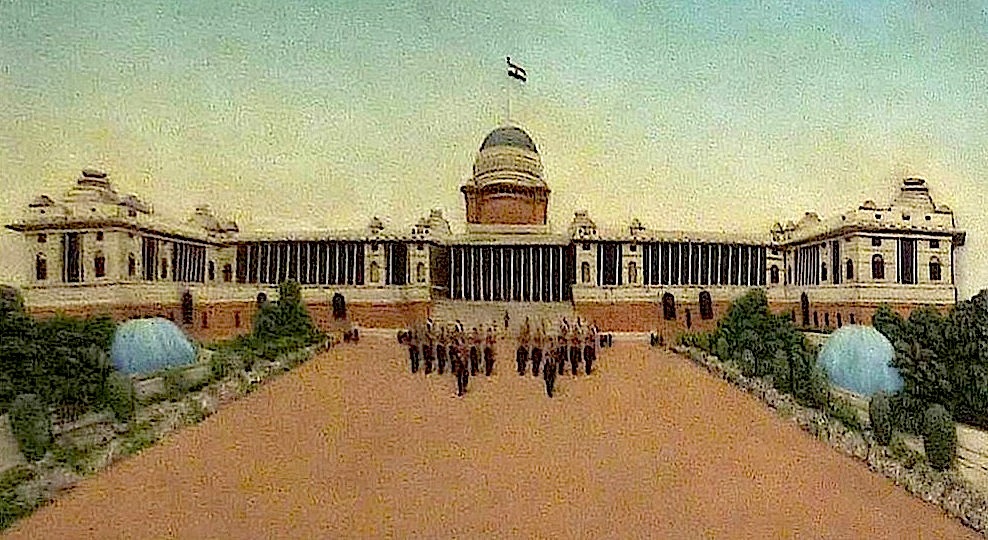The image appears to depict a highly detailed and possibly digitally altered or illustrated scene of a grand government building, likely a capital or palace. The foreground features a light beige pathway flanked symmetrically by greenery, such as green bushes and perhaps a bluish mound that might be a rock or decorative element. The pathway leads up to wide steps that access the main building, which stretches horizontally with impressive vertical columns in black and white. The central structure of the building is capped with a grey dome, adorned with a flag that appears to have brown, white, and green colors—though the exact hues are unclear due to the grainy quality of the image.

In front of this majestic structure, within the courtyard, a couple dozen dark-clad individuals are lined up, suggesting a military formation or some formal assembly. Their precise uniforms are hard to distinguish, but the overall dark color is noticeable. The sky above the scene is a mix of blue with a brownish tint near the horizon, perhaps indicating a smoggy atmosphere. The entire scene, despite being potentially pixelated or heavily stylized, showcases an intricate attention to detail in both architectural and natural elements.